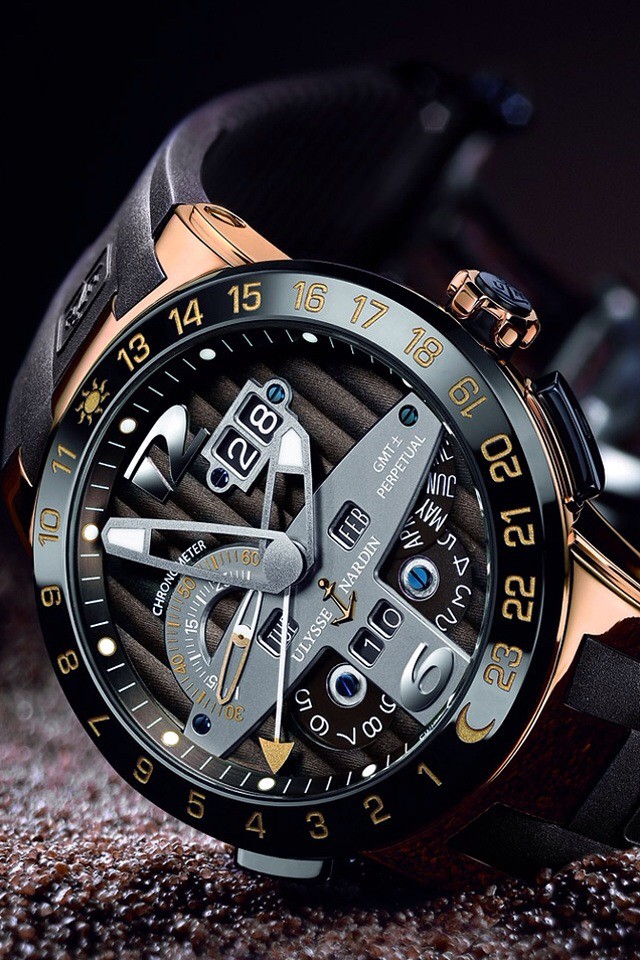This image features a luxurious wristwatch placed on a bed of red gravel. The watch boasts an elegant black wrist strap and a striking face adorned with copper and black elements. A diamond accent adds a touch of opulence. The dial displays a full array of numbers encircling the face, while the top portion is illuminated by sunlight and the bottom by moonlight, providing a day-night indicator. The hour hand points between 15 and 16, with the minute hand nearing the 10-minute mark. Additionally, a smaller window on the bottom right showcases the date "February" and the day "Tuesday." A prominent numeral six sits at the bottom of the face, completing the sophisticated design of this intricate timepiece.